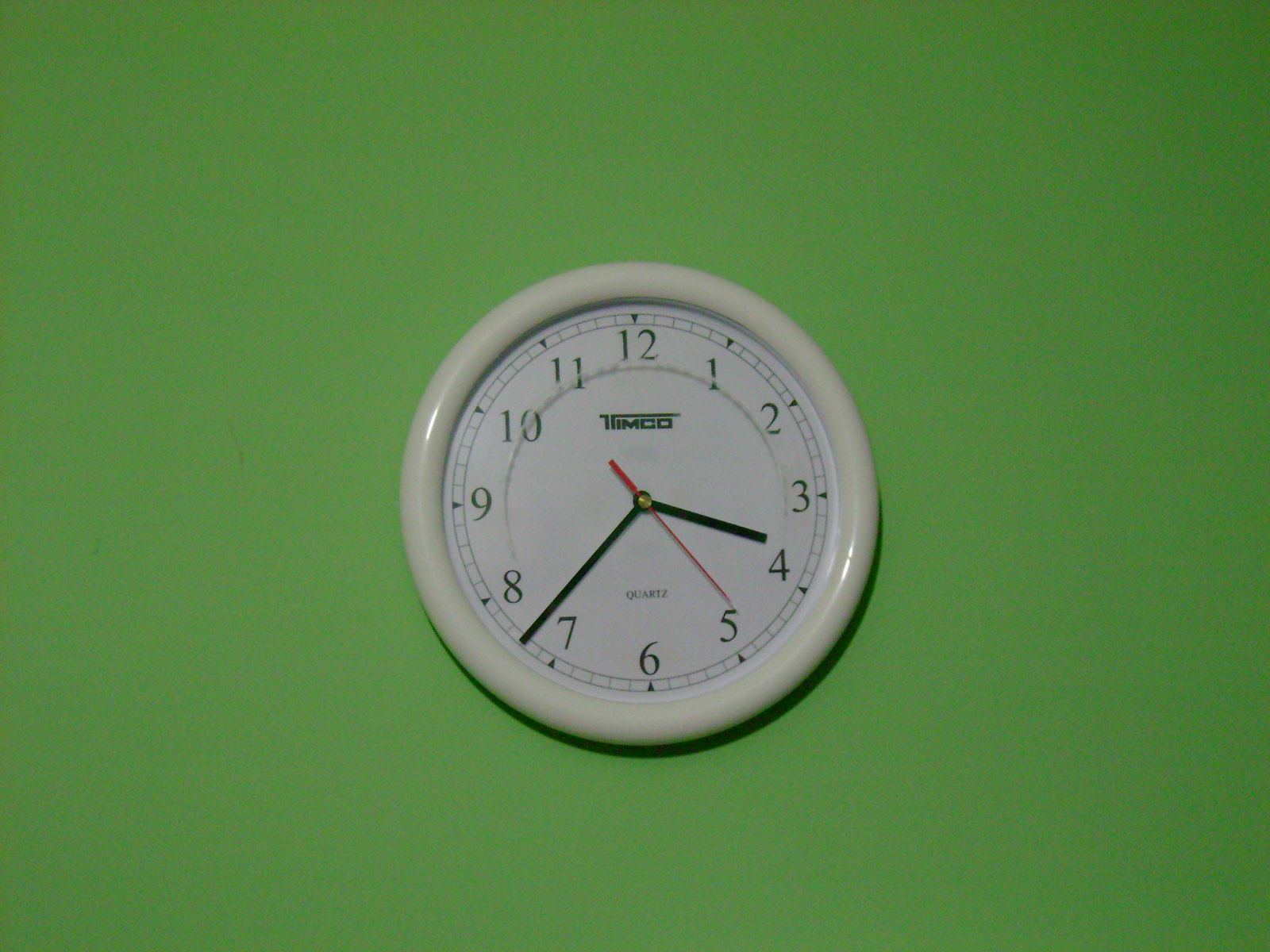This image features a simple yet detailed wall clock against a medium green background, darker than lime but lighter than hunter green. The clock stands out with its white face and rounded, reflective plastic bezel. Standard Arabic numerals from 1 to 12 encircle the face, each accompanied by a small black triangle. At the 12 o'clock position, the brand name "Timco" (T-I-M-C-O) is printed in black, and just above the 6 o'clock position, the word "Quartz" (Q-U-A-R-T-Z) is also noted in black. The clock's hour and minute hands are thin, black sticks, while the second hand is red. The time displayed is 3:37 and 24 seconds.